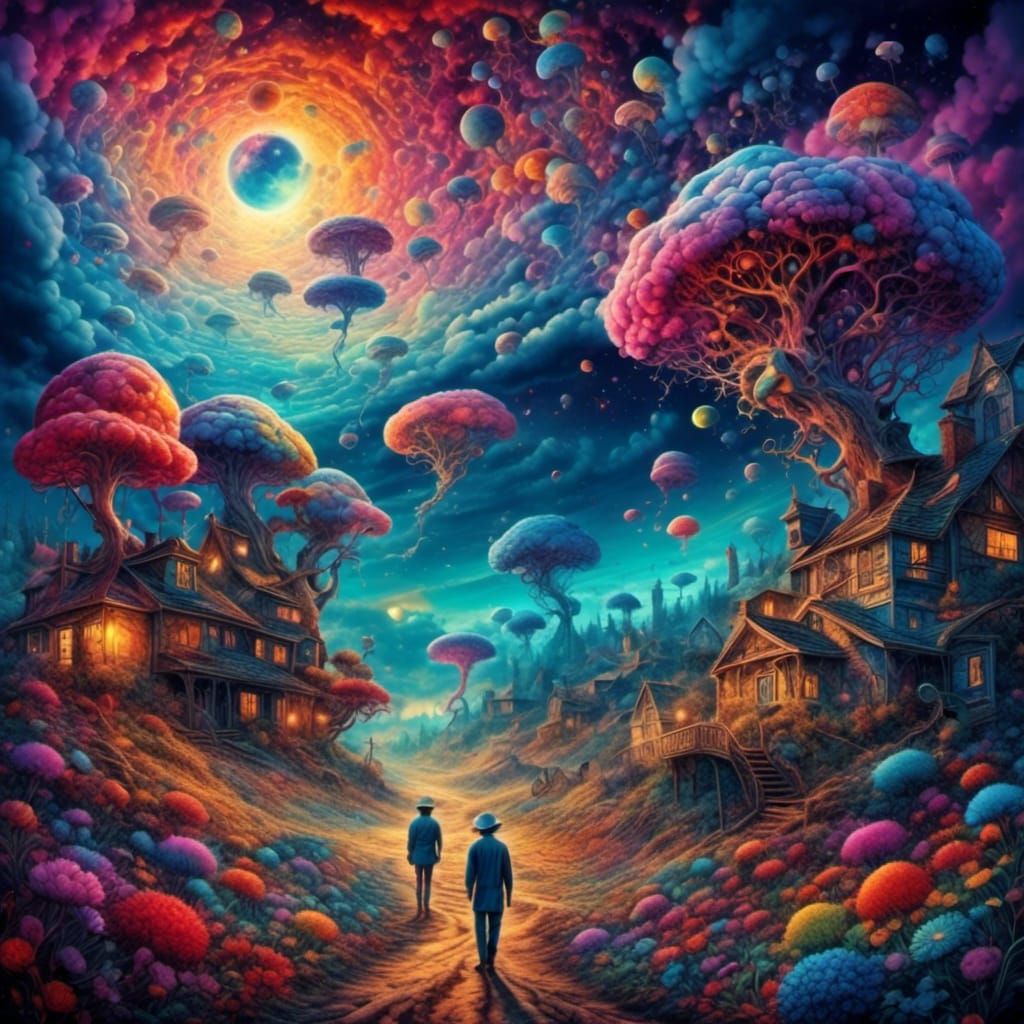The image is a vibrant and fantastical illustration, seemingly AI-generated. It features two people, each wearing a white hat, walking along a dirt path lined with wildly colorful flowers that resemble edible treats and echo the fantastical nature of the scene. On either side of the pathway are multi-story wooden houses with steep gabled roofs and glowing windows, each hosting trees that appear to grow organically through them. These trees have branches that look twisted and intervolved, culminating in bright, cotton candy-like florets of magenta, blue, turquoise, orange, yellow, and purple.

Above this surreal landscape, the sky is filled with dark blue and turquoise clouds forming a vortex that blends into a gradient of blue, purple, and orange, potentially surrounding a planetary or solar eclipse. Floating like balloons, more cotton candy-like trees drift upwards, creating a whimsical and otherworldly environment. The vivid use of color and imaginative elements, such as the floating trees and their cauliflower-like structure, along with the detached, interwoven branches, contribute to an overall dreamy and fantastical atmosphere.